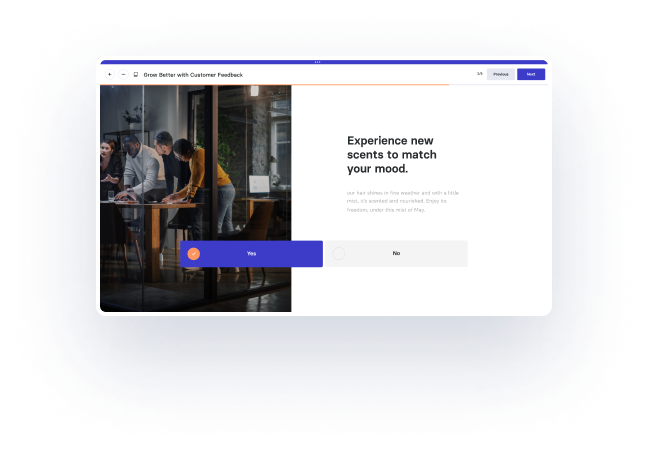This image captures a minimized photograph of a webpage, shrunken to the size of a thumbnail. The top section of the webpage features a white background, with a blue bar that extends partially off-screen. Immediately below, in a prominent black font, is the text "Grow better with customer feedback." To the right of this text are a refresh button and a forward button.

Further down, two interactive buttons are partially visible: one labeled "Proceed" and the other "Join," with "Join" highlighted in blue. A large photograph dominates the right side of the page, depicting four people gathered around a table in an office setting. They appear to be engaged in conversation, all looking down at some focal point.

On the left side, a segment of the webpage displays the headline "Experience new scents to match your mood" in large black font. Below this headline is a paragraph providing additional details, though the specifics are not entirely clear in the image. Toward the bottom of the screen, two prominently placed, large rectangular buttons are visible: the button on the left, labeled "Yes," is highlighted in blue, indicating it has been selected, while the button on the right, labeled "No," remains in grey.